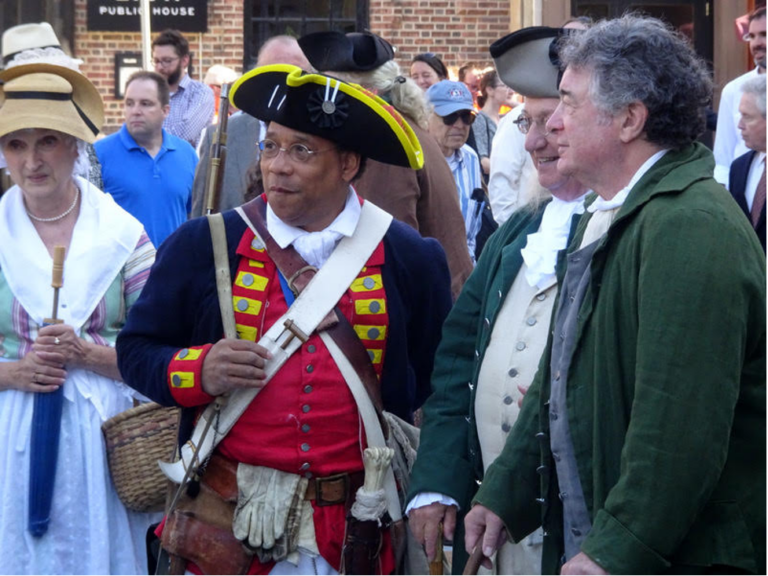In an outdoor setting reminiscent of Colonial Williamsburg, the image captures a historical reenactment with four individuals in the foreground dressed in American Revolutionary-era clothing. On the far left, a woman dons a green, purple, and white dress, complemented by a tan hat with a black bow, and holds a closed blue umbrella. Next to her stands a man in a captain's uniform, featuring a black tricorn hat with yellow trim, a red vest, and a blue jacket adorned with red and yellow squares. He also has wire-rimmed glasses and wears a white and brown strap across his shoulders, with gloves tucked into his belt. Flanking him are two men in long green jackets with white shirts that have frilly sleeves, each sporting black tricorn hats, embodying the colonial aesthetic. Behind these reenactors, spectators in modern attire, such as polo shirts and hats, observe the scene. The backdrop includes a brick wall with windows and a black sign with white lettering that reads "Public House," enhancing the historical ambiance. The vibrant palette includes shades of white, yellow, red, blue, green, purple, tan, and black.